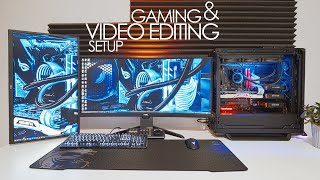The image showcases a detailed and sophisticated "Gaming and Video Editing Setup" as indicated by the text at the top center. The setup consists of two monitors: a horizontal widescreen monitor centrally located, and a vertically oriented monitor to the left, both displaying a blue futuristic pattern. A long, rubber-like desk pad stretches across the foreground, accommodating a lit-up keyboard on the left and a black mouse on the right. To the right of the central monitor is a sleek, black-framed desktop computer tower with a transparent side panel that reveals glowing blue and red internal components. The setup sits on a flat, white table surface. Behind the arrangement, black window blinds provide a contrasting backdrop, and a small plant adds a touch of green to the right of the computer tower. Further enhancing the ambiance, foam-ridged sound dampening pads line the white wall behind the setup, creating a focused and immersive environment perfect for gaming and video editing.